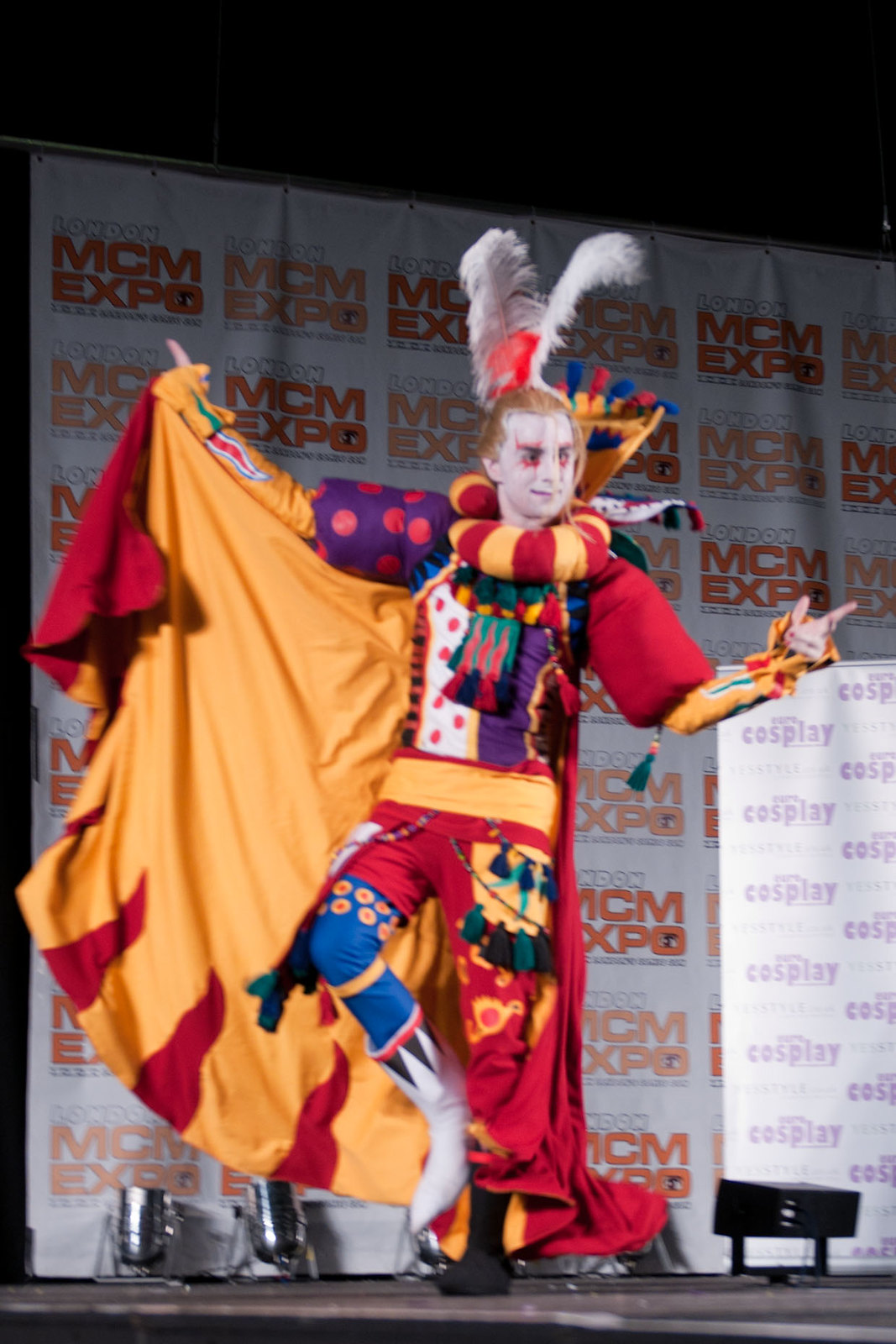The image depicts a person dressed in an elaborate, colorful costume, reminiscent of a festive clown or jester, perhaps an anime character. His face is painted white with red war paint around the eyes, and blonde hair partially covers his face. The vibrant costume includes a red left shoulder pad, polka dot right shoulder pad, and a red and yellow-striped scarf around his neck. He sports a yellow belt adorned with small bags and tassels, multicolored pants – red on one side and blue on the other – and mismatched boots, one black and one white. He holds up a yellow and red cape with one hand, with large feathers protruding from behind his head, suggesting a dynamic, mid-dance pose. The setting appears to be a stage at the London MCM Expo, with a backdrop featuring 'Cosplay' in purple letters, illuminated by stage lights.